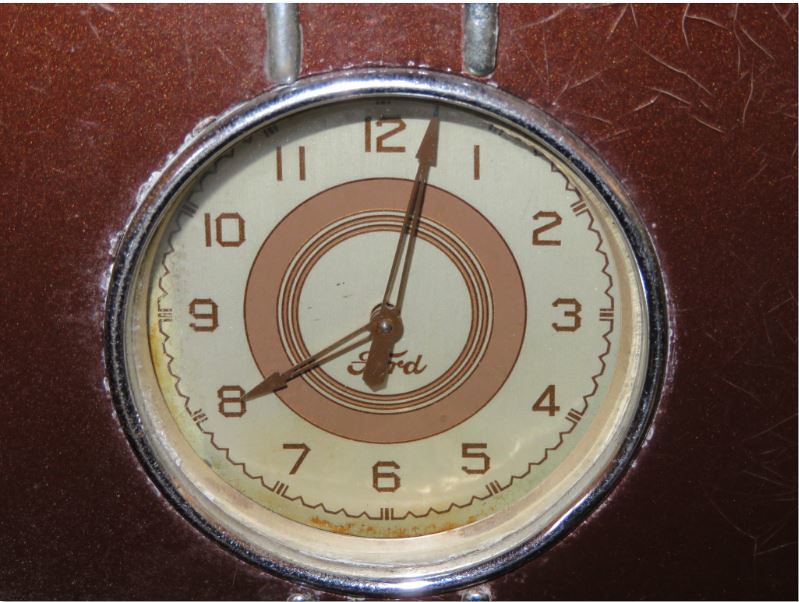This photograph features a vintage clock with a distinct retro aesthetic. The clock is encased in a silver metal border, with two vertical silver lines extending from the top, adding to its old-fashioned charm. The backdrop is a maroon gradient, transitioning from a lighter hue above to a deeper shade below, adorned with numerous scratches that speak to its age and history. 

The clock face itself is a heavily faded blend of yellow and off-white, lending a sense of antiquity. The numbers on the clock are inscribed in a dark brown font, which contrasts with the worn-out background. At the center of the clock face, there is a circle featuring alternating lighter and darker brown stripes, creating a focal point. 

The clock's hands, both in dark brown color, are positioned to mark the time: the shorter hand pointing just past the 12 and the longer hand aimed at the 8, indicating a time of approximately 1:40. The hands, slightly raised, add a three-dimensional aspect to the clock's vintage look.